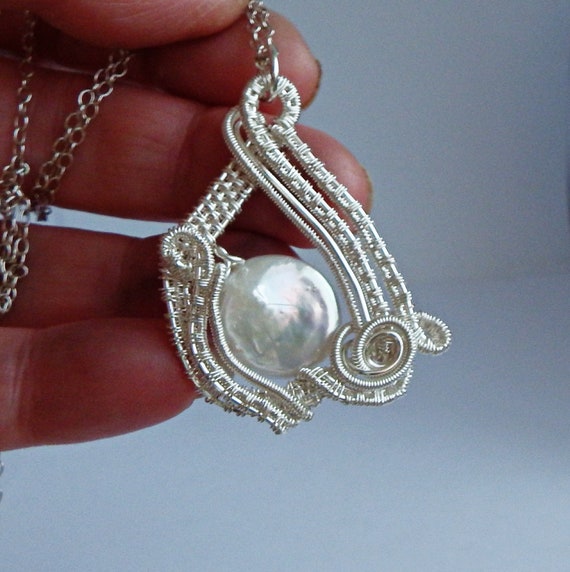In this detailed close-up photograph, a woman with darker skin tone fingertips holds a unique, possibly handmade piece of jewelry against a light blue-gray background. The silver-toned chain, thick and intricately designed, wraps around her middle, ring, and pinky fingers, showcasing its elegant loops and swirls. The pendant, prominently positioned, features elaborate silver wiring that twists and turns, enclosing a lustrous white pearl at its center. The background, adding a subtle contrast, allows the bright silver of the pendant to stand out, highlighting the craftsmanship and delicate details of the swirling silver frame that beautifully holds the medium-sized pearl.